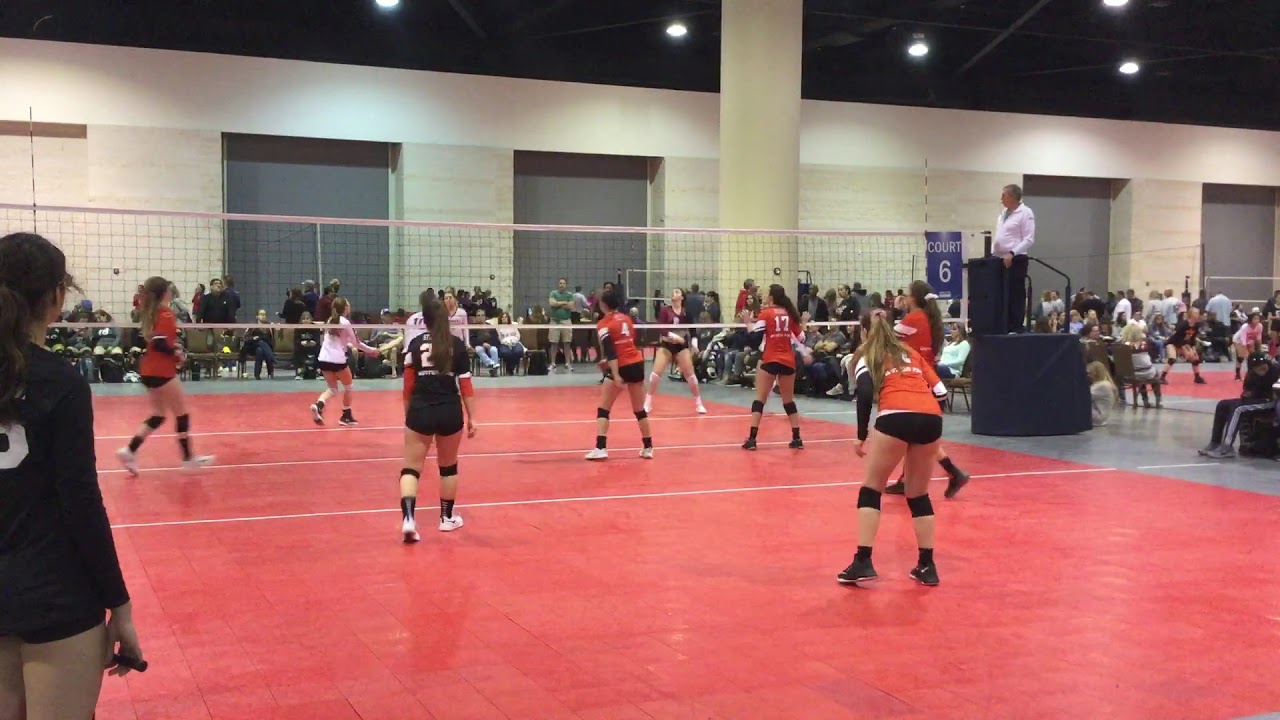This vibrant, horizontally aligned rectangular photograph captures an intense indoor girls' volleyball game at a busy recreational center, possibly during a tournament given the abundance of spectators. In the foreground, the main court, with its red-tiled surface bordered by gray tiles, is the focal point. One team, clad in striking orange jerseys and black shorts, are fully engaged in the game, their black knee pads adding to their uniformity. The opposing team sports white shirts paired with black shorts. 

Positioned in the far left corner, a player in a black jersey, only partially visible, stands with her back to the viewer, her long brown hair cascading down and a number visible on her back. A centrally-placed white net divides the court, with a referee in a white long-sleeved shirt and black pants overseeing the match from an elevated black platform. 

The background reveals more details, including a crowd of spectators seated on benches or chairs against white walls accented with large, square gray areas, reminiscent of potential garage door openings. Overhead, the black ceiling with recessed lighting ensures the court is well-lit. In the top right corner, another volleyball net hints at multiple games occurring simultaneously, underscoring the vibrant, competitive atmosphere of the setting.